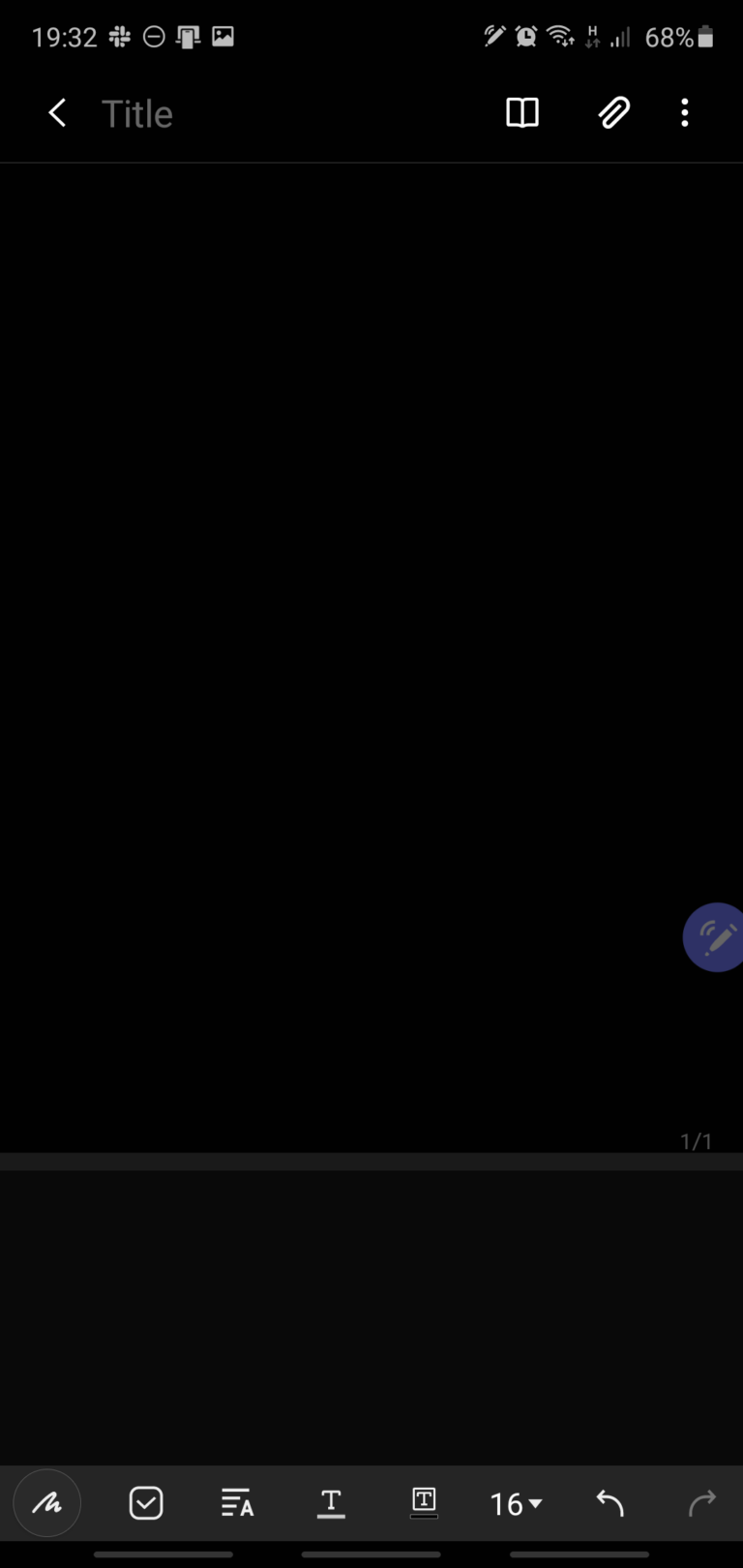A detailed caption for the described image could be:

"This image, captured from a cell phone screen, features a predominantly black background. At the top of the screen, the time '19:32' is displayed prominently. To the right of the time, there are four clickable icons. On the opposite end, near the battery icon displaying '68%', there are five additional clickable icons. Below this top bar, a left-pointing white arrow precedes a gray text labeled 'Title'. Further down, graphical elements depict an open book or two pages of a book, followed by a paper clip icon, indicating an attachment feature, and a vertical ellipsis (three vertical dots) for more options. Towards the lower-middle section of the screen, a faint gray line extends horizontally from the left to the right edges. Situated along this line, the text '1 of 1' appears, alongside a partially visible, bluish pen icon, slightly cut off at the right edge of the screen. At the very bottom, additional icons are present, enhancing the functionality provided through the interface."